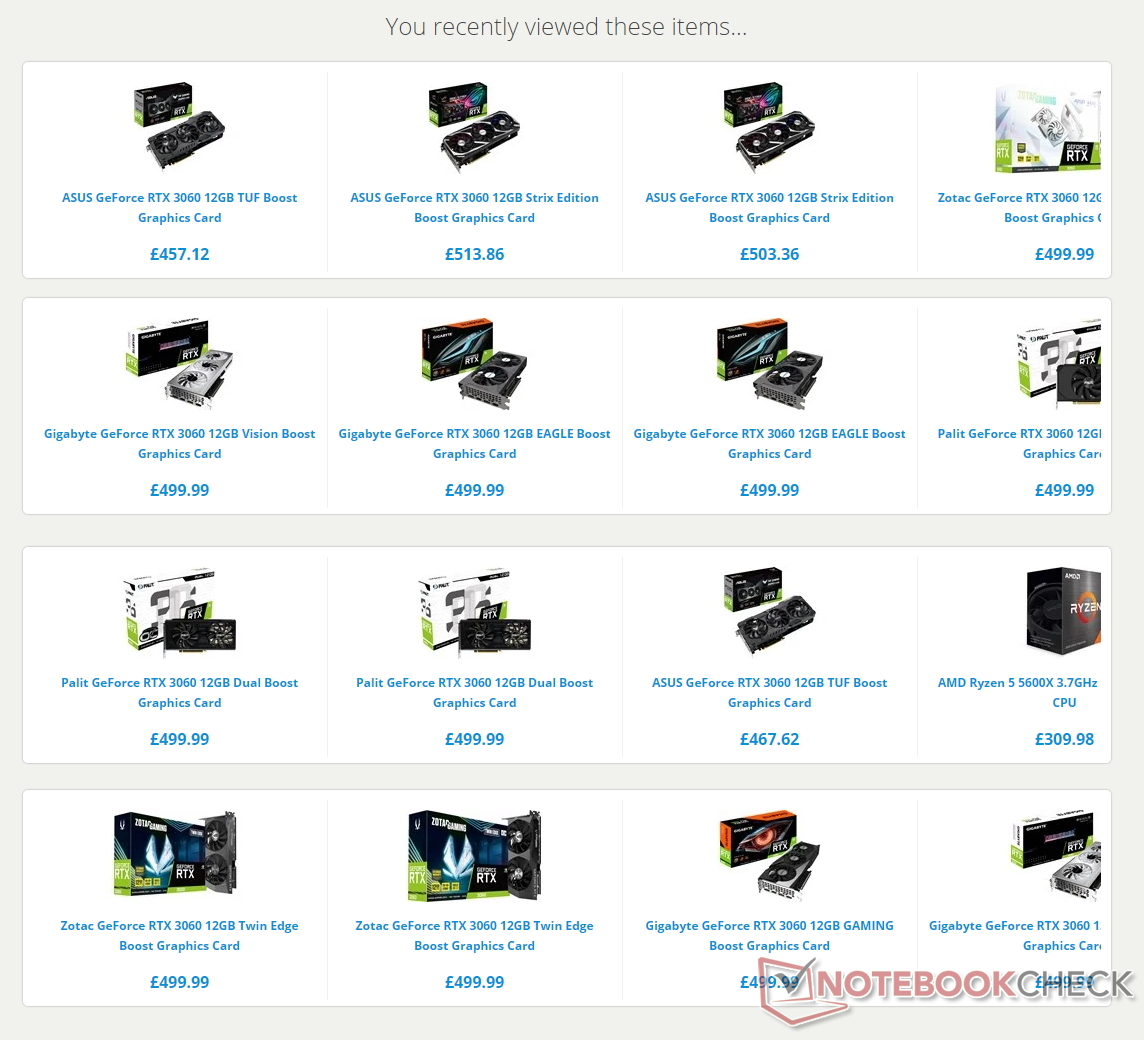A screenshot of a webpage displays a "Recently Viewed Items" section featuring four rows of high-end graphics cards. Each card is priced around 500 British pounds. The first product listed is an Asus GeForce RTX 3060 with 12 gigabytes of memory, labeled as a "Toughboost" graphics card. The image conveys that all the graphics cards share similar specifications but vary in branding and slight feature differences, such as "Dual Boost" and "Twin Edge." This selection provides a comprehensive comparison for those interested in the detailed specifications and nuances of each card.